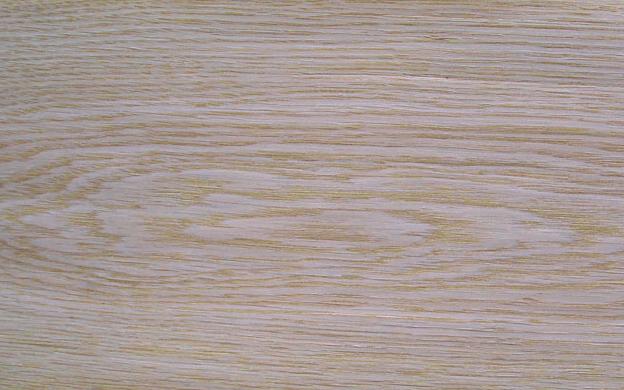The image showcases a close-up of a wooden surface, possibly a plank, with intricate wood grain patterns. The wood itself has a light brown hue, accented with slightly darker, medium brown circular patterns at its center. These concentric rings are prominent from left to right in the middle of the image. As the pattern extends towards the top and bottom edges, these circles transition into straight, horizontal grain lines. The surface appears to have no writing or objects, purely emphasizing the natural beauty of the wood grain. Additionally, the texture of the wood is somewhat ripple-like, reminiscent of gentle ocean waves, and interspersed with occasional white streaks that add to its visual complexity. The light brown wood might also have a subtle violet tint, giving it a unique, faded purplish background color that contrasts with the brown swirls.